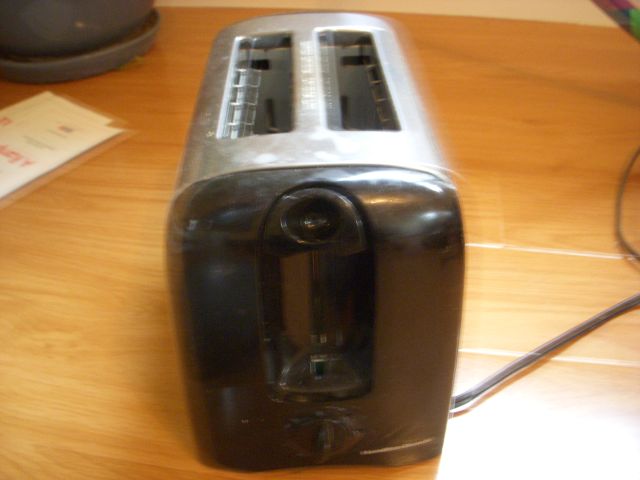In the image, a worn and scratched toaster sits prominently on a brown wooden table. The toaster, which features a black plastic side face and a silver metal body, is oriented so that the viewer can see its edge directed towards the upper middle part of the frame. The device has two slots for bread and appears to be quite old or possibly broken. A black cord extends from below the toaster, trailing off to the right.

To the left of the toaster, there are two pieces of paper, stacked one on top of the other. In the upper left corner of the image, part of a dark gray planter pot with a tray, sitting on the table, is visible. Something indeterminate rests in the tray part of the planter. The background includes a partial view of a beige wall at the very upper part and to the right of the image. No bread or toast occupies the toaster at the moment, and the lever and dial are clearly visible on its front.